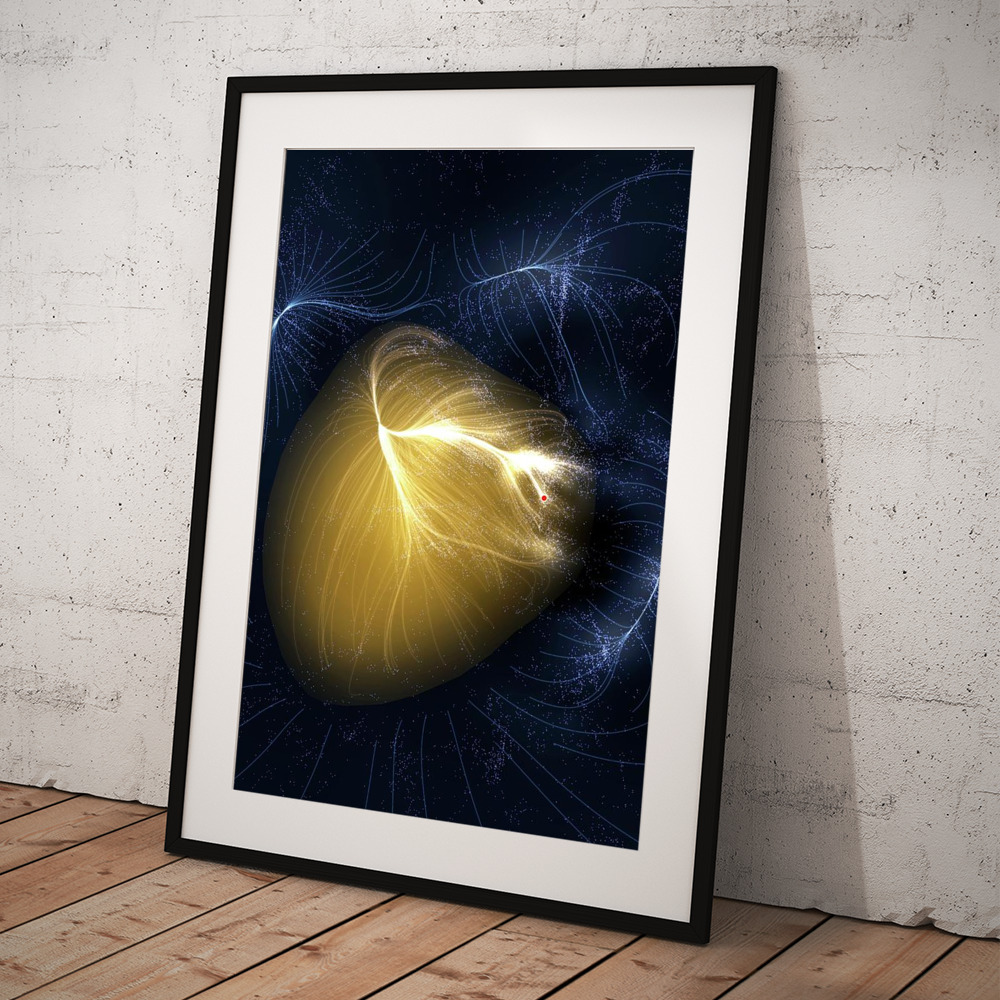The image is a detailed artwork displayed in a black frame with a white mat, propped against a white masonry wall. It's situated on what appears to be an unfinished pine floor. The artwork itself features an abstract, feathery, or jellyfish-like underwater creature glowing in a yellow-gold color, accompanied by similar filament-like structures glowing white. These luminescent forms are set against a backdrop that appears black or deep blue, almost suggesting currents of electricity or luminous paths. In the center of the image, there is a prominent golden structure with two illuminated gold lines and a red dot at one end, enhancing its ethereal quality.